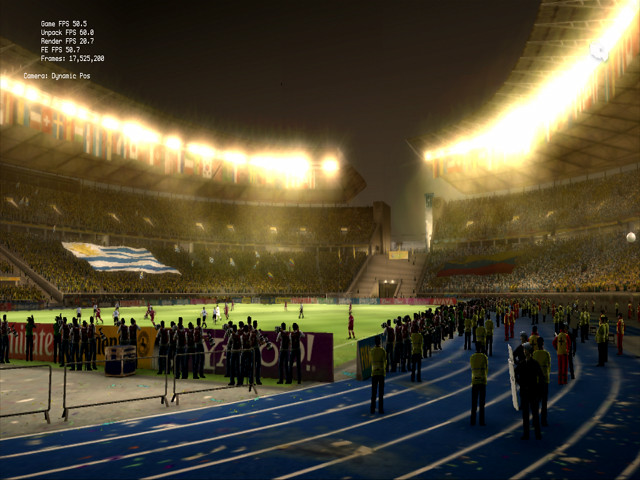The image is a snapshot from a video game displaying a stadium scene. At the top of the image, a white font overlay provides game performance metrics such as frames per second and other statistics. The stadium is brightly illuminated by mounted lights on a metal structure. The stands are packed with spectators who are waving flags from two countries. To the left, fans are holding up a flag featuring gold, white, and blue colors. On the right, the flag is yellow, blue, and red. Spectators dressed in yellow, dark, and red attire stand on a blue track-like surface, while others are positioned on the grass. Players are actively engaged in a game on the field. Behind some advertising signage, more spectators can be seen watching the action.